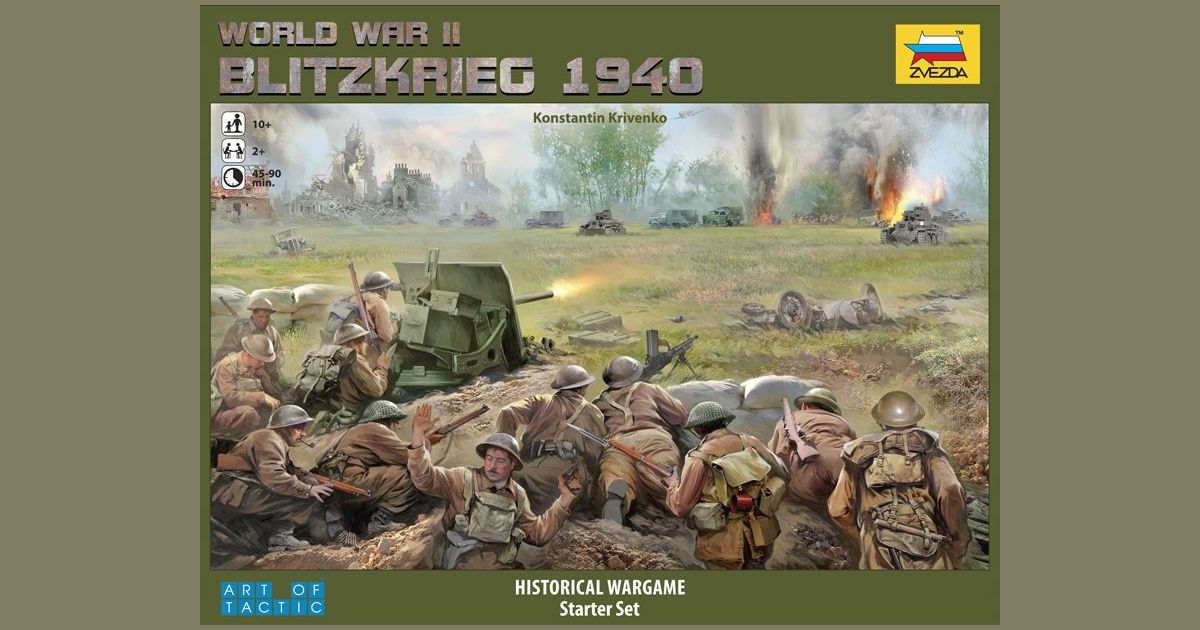This image showcases the box art of a World War II-themed board game titled "World War II: Blitzkrieg 1940." Dominating the center of the image is a war scene, intricately detailed with soldiers in brown uniforms and metal helmets. These soldiers are either sitting or lying on the ground, engaged in combat. They are depicted firing their weapons amidst a battlefield dotted with burning army vehicles, white smoke billowing from the fires, and a grassy terrain. 

The top of the image features a dark green horizontal strip with the game's title, "World War II: Blitzkrieg 1940," prominently written in white. On the top right corner, within a yellow rectangle, is the logo "Zvezda" next to a flag, identifying the game's publisher. At the bottom, another green horizontal strip contains two main elements: on the left, the words "Art of Tactic" in turquoise blue letters, and in the center, "Historical War Game Starter Set" in white text. Additionally, the image has two gray vertical strips on the left and right sides, framing the central war scene, providing a structured border to the box art. This game is suitable for players aged 10 and above.